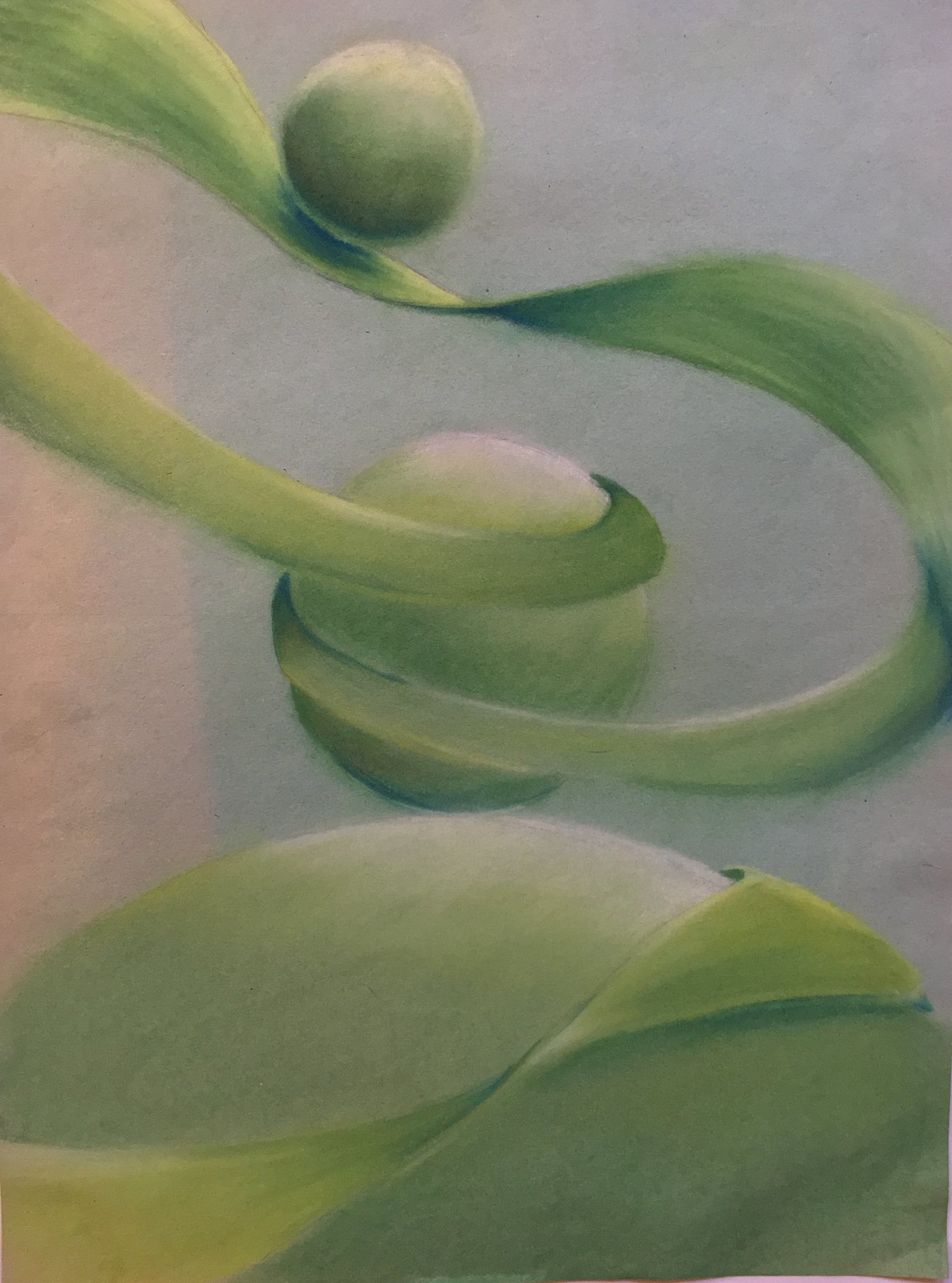A detailed watercolor painting features a collection of three green orbs arranged from the foreground to the background against a light blue backdrop. In the foreground, the upper portion of a large green orb is prominently displayed. A smaller green orb resides in the center of the composition, while the third green orb is partially visible, emerging from the upper left corner of the painting. 

Intertwining diagonally across the scene is a delicate, green ribbon. This ribbon threads beneath the partially visible orb at the top left, loops to the right, then elegantly curves down along the right edge before re-entering the frame to loop in front of the central orb. It wraps around the central orb and continues to loop up to the left, eventually exiting the frame.

In the foreground, another green ribbon enters from the lower left corner and arches over the large, partially visible orb. This ribbon twists as it extends diagonally to the right, tucking behind the orb before disappearing from view. 

The overall coloring of the painting is soft and subdued, with the ribbons and orbs rendered in light green tones, accentuated by subtle shading on their bottom left sides. The background is a gentle, pale blue, creating a serene and ethereal atmosphere. The image is devoid of any textual elements, allowing the viewer to focus solely on the fluid and harmonious interplay between the orbs and ribbons.